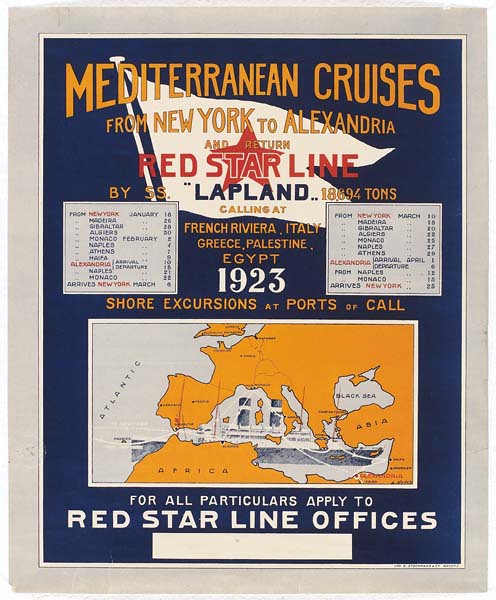This vintage poster advertisement, framed by a gray border, promotes Mediterranean cruises offered by the Red Star Line aboard the S.S. Lapland, a 18,694-ton vessel. Bold orange lettering at the top announces "MEDITERRANEAN CRUISES" in all capitals, with a subtler curved text beneath stating, "From New York to Alexandria and Return." Key destinations include the French Riviera, Italy, Greece, Palestine, and Egypt, with the year marked as 1923. Nestled within the design, there is an iconic red star symbol synonymous with the Red Star Line. Flanking the central text are two side boxes detailing the itinerary, such as departures from New York on March 10th and arrivals in Naples on March 17th. Below the text, a yellow-and-white map spans Europe and North Africa, highlighting the cruise route through Asia, Africa, and near the Black Sea. Each segment of the journey is illustrated, emphasizing short shore excursions at various ports of call. At the bottom, the poster instructs interested travelers to "For all particulars apply to Red Star Line offices."